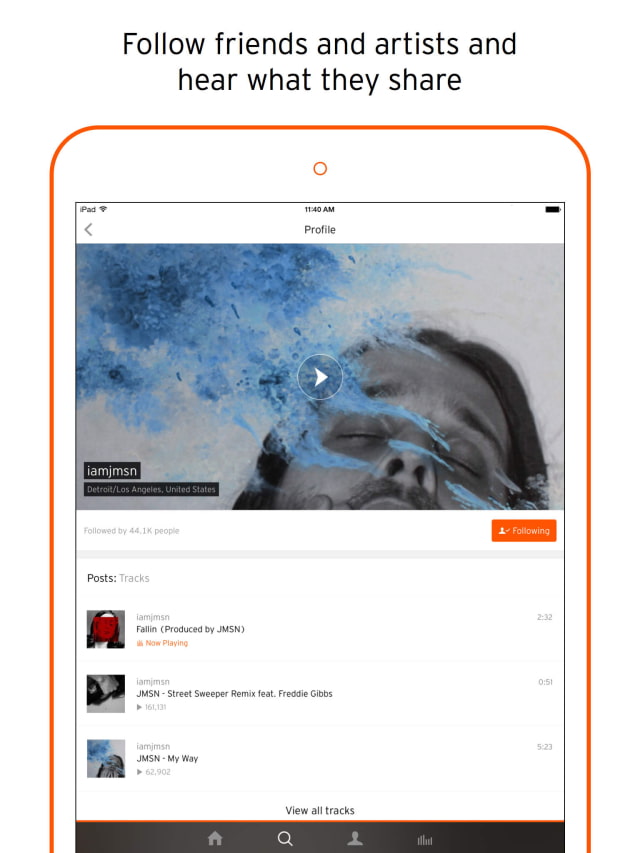The image showcases a mobile interface on a white background with key elements detailed as follows:

In the center of the image, black text reads "Follow friends and artists and hear what they share." This text is enclosed within an orange-outlined circle. Just below this circle, the time "11:40 a.m." is displayed.

On the top of the image, the word "iPad" is positioned above a gray arrow pointing left. On the right side, there is a battery logo indicating the device's charge level. 

Further down, an image with a blue background features a person’s face in gray. This image includes a white arrow inside a white circle, suggesting a play button.

To the left of this image, within a black box, white text reads, "I am JMSN." On the right side, an orange box with white font states, "Following."

Below these buttons, the text "Post..." appears, likely indicating an unfinished or truncated title. The next line reads: "Faith (produced by JMSN)." Following this, the text "JMSN Street Sweeper Remix featuring Freddie Gibbs" appears. Another line lists "JMSN - My Way."

Towards the bottom of the interface, a centered option in black font reads "View all tracks." The bottommost section features a black bar with four grayish icons arranged from left to right: a house, a magnifying glass, a person, and a set of lines going up and down, representing different navigation options on the app or website.